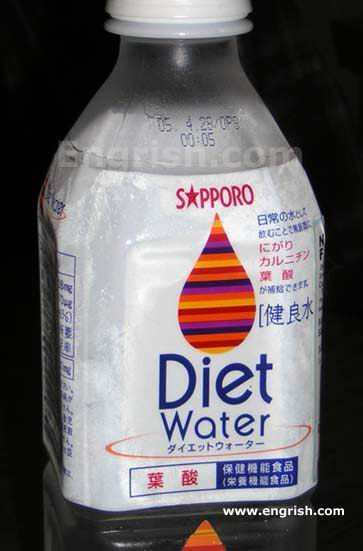The image is centered around a water bottle set against a stark black background, drawing focus exclusively to the bottle itself. The bottle cap is white, matching the label that wraps around its side. The label displays several pieces of text: starting from the top, it reads "05.4.28.0ps." Directly below this, the numbers "00, 05" are printed. Additionally, above the main section of the label, there is a single letter "S." A star surrounds the text "PPORO." In the bottom right corner of the image, the website URL "www.engrish.com" is visible in white font. The simplicity of the background accentuates the details on the water bottle, making them the focal point of the image.